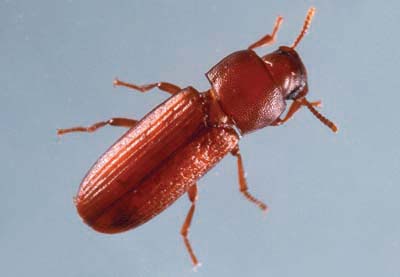This is a high-resolution close-up photograph featuring a reddish-brown beetle, likely a flower beetle, standing on a light blue or grayish surface. The beetle's body is elongated with a distinct red head, thorax, and midsection, all covered by a matching exoskeleton. Its two prominent, non-damaged antennae and six legs are also evenly reddish in hue. The image shows an aerial view, capturing the beetle facing toward the top right corner. The beetle's hind legs appear longer, suggesting it's possibly closer to the viewer. Despite some compression artifacts that introduce slight blurriness and noise, the beetle's detailed segmentation - including the head, thorax, and wing casings - remains visible.